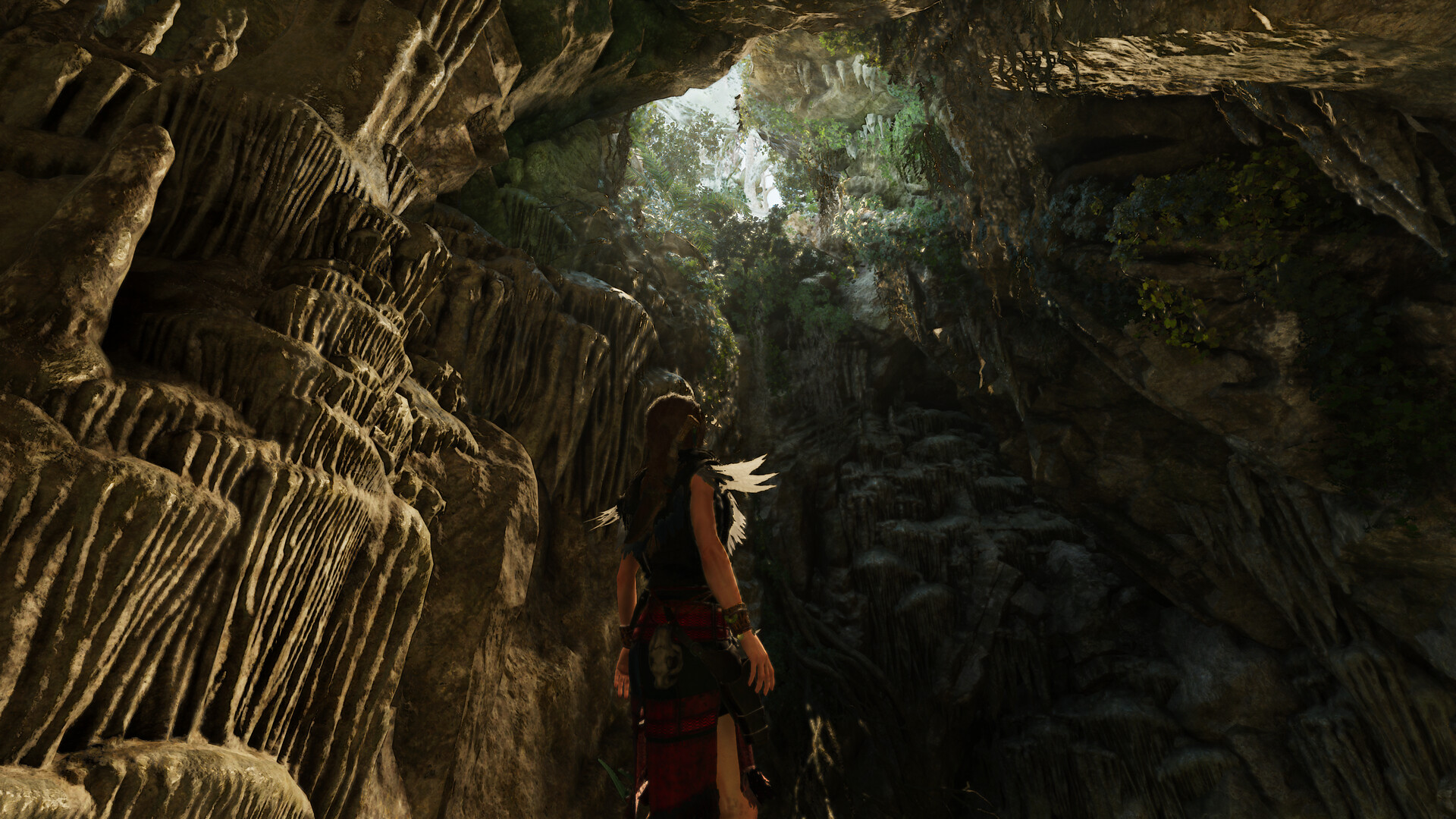The image appears to be a scene from a video game, depicting a detailed and atmospheric cavern. On the left side of the image, there are intricate, indented cavernous falls, crisscrossed by lines running vertically and horizontally. The rock wall in the background is rugged and folded, resembling a series of natural bridges. At the top of the cavern, an opening reveals a glimpse of the sky and some green foliage, adding a touch of nature to the rocky environment.

To the right, the cavern walls are slightly damp, adding to the sense of realism and immersion. In the foreground, a character is standing prominently. The character is adorned with a wrist bracelet and has feathers around their neck. They appear to be wearing a dress, adding a touch of cultural or historical detail to the scene. The overall composition blends natural and fantastical elements, highlighting the intricate design typical of immersive video games.